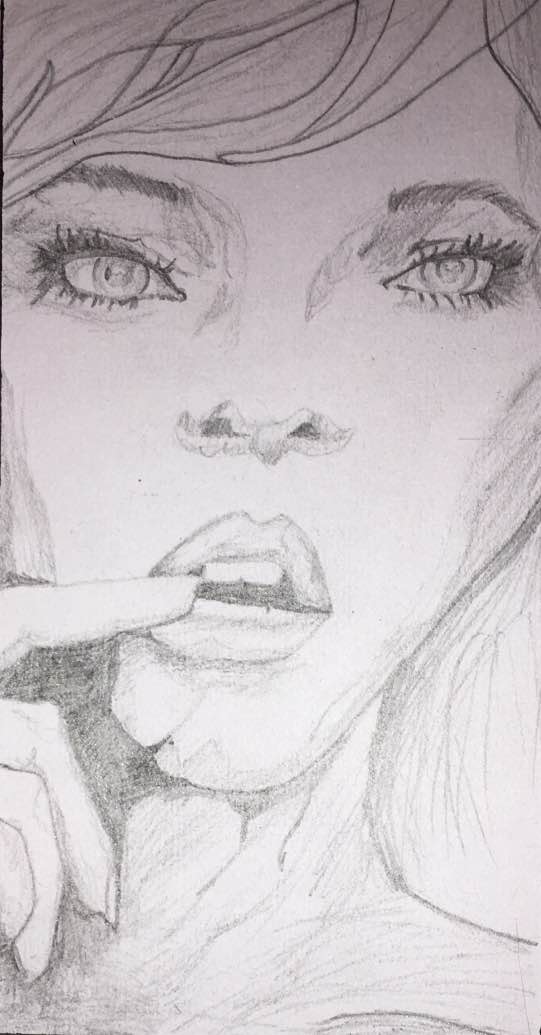A detailed portrait drawing of a woman dominates the frame, capturing her in a seductive pose. The woman’s face occupies nearly the entire length and width of the image, with the top and sides of her head extending beyond the borders of the picture. Her captivating eyes, seemingly light in color, are accentuated with thick, clumpy mascara on both the top and bottom lashes. Her meticulously groomed dark eyebrows frame her eyes, lending an intense focus to her gaze.

Her flowing hair falls delicately across her forehead, partially obscuring her bangs. The drawing depicts her wearing heavy eye makeup, which adds to the pronounced effect of her alluring expression. Her slightly open lips, lined with lip liner and possibly filled with lipstick, reveal her two front teeth. A single finger gently touches her lower lip, enhancing the seductive nature of her pose.

The portrait also captures the contours of her neck and the bare expanse of her shoulders, suggesting a possible state of undress. Overall, the drawing expertly conveys a sense of beauty and allure through detailed facial features and an evocative pose.